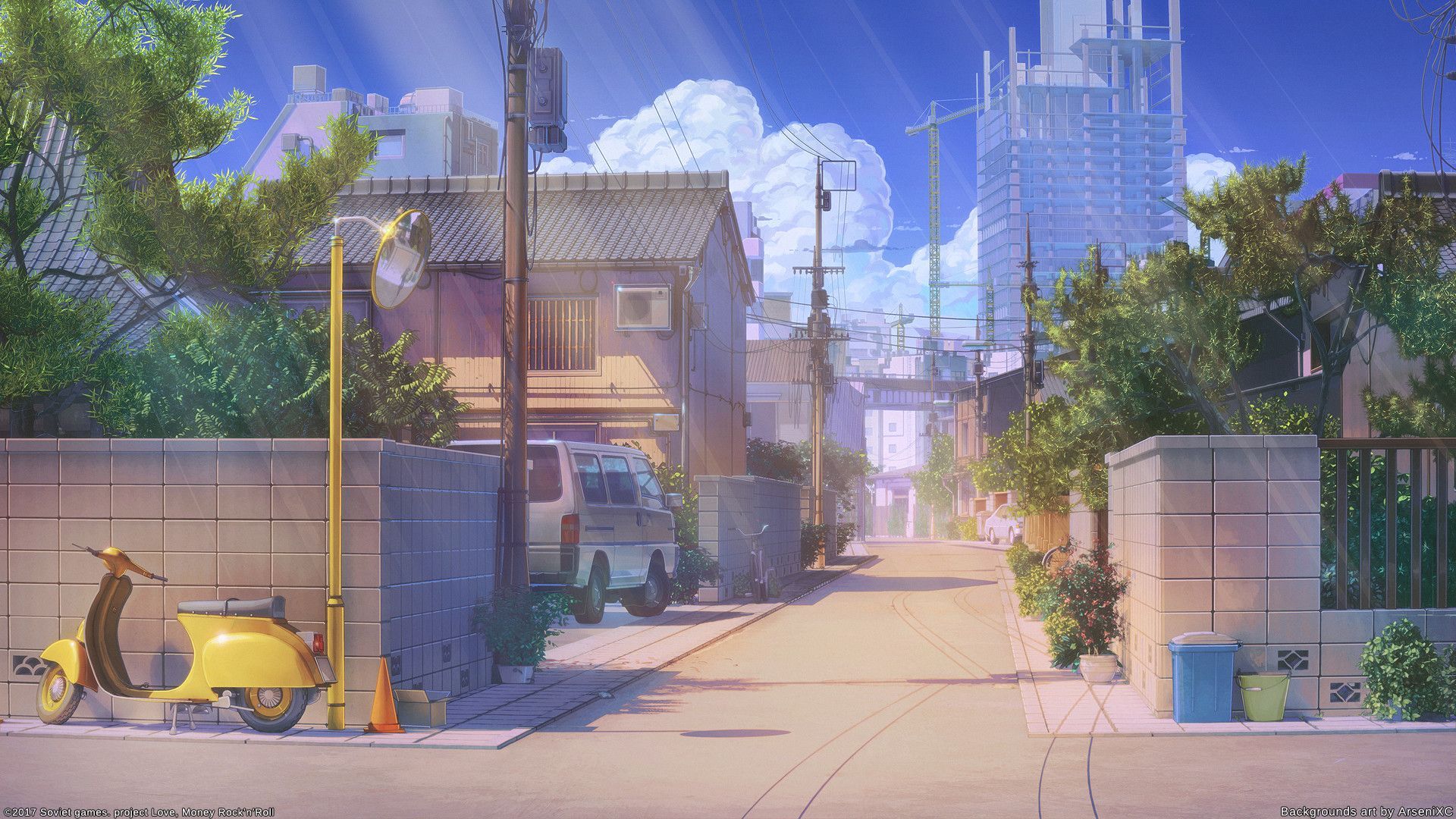This detailed digital 3D image captures a vibrant city street scene, rendered with precision and color. The foreground features a brown-colored roadway flanked by a cinder block wall and brick pillars just before the entrance of a driveway. On the left side, we see a yellow scooter parked beside a street lamp, and further back, a rust-colored house with a gray roof stands alongside a green bush and tree. A brown and silver van is parked in the driveway next to the house. The house also features an air conditioner on an upper level window. To the right side of the street, another green bush sits next to a blue trash bin and a green bucket, resting near a large blue and gray skyscraper in the background. Utility poles and additional buildings, including a pink building and a teal box-like structure with a window, can be seen further back. Above, the sky is a bright blue filled with fluffy white clouds, with beams of sunlight adding a serene glow to the entire scene. Cranes surround a tall skyscraper under construction, enhancing the dynamic urban atmosphere.